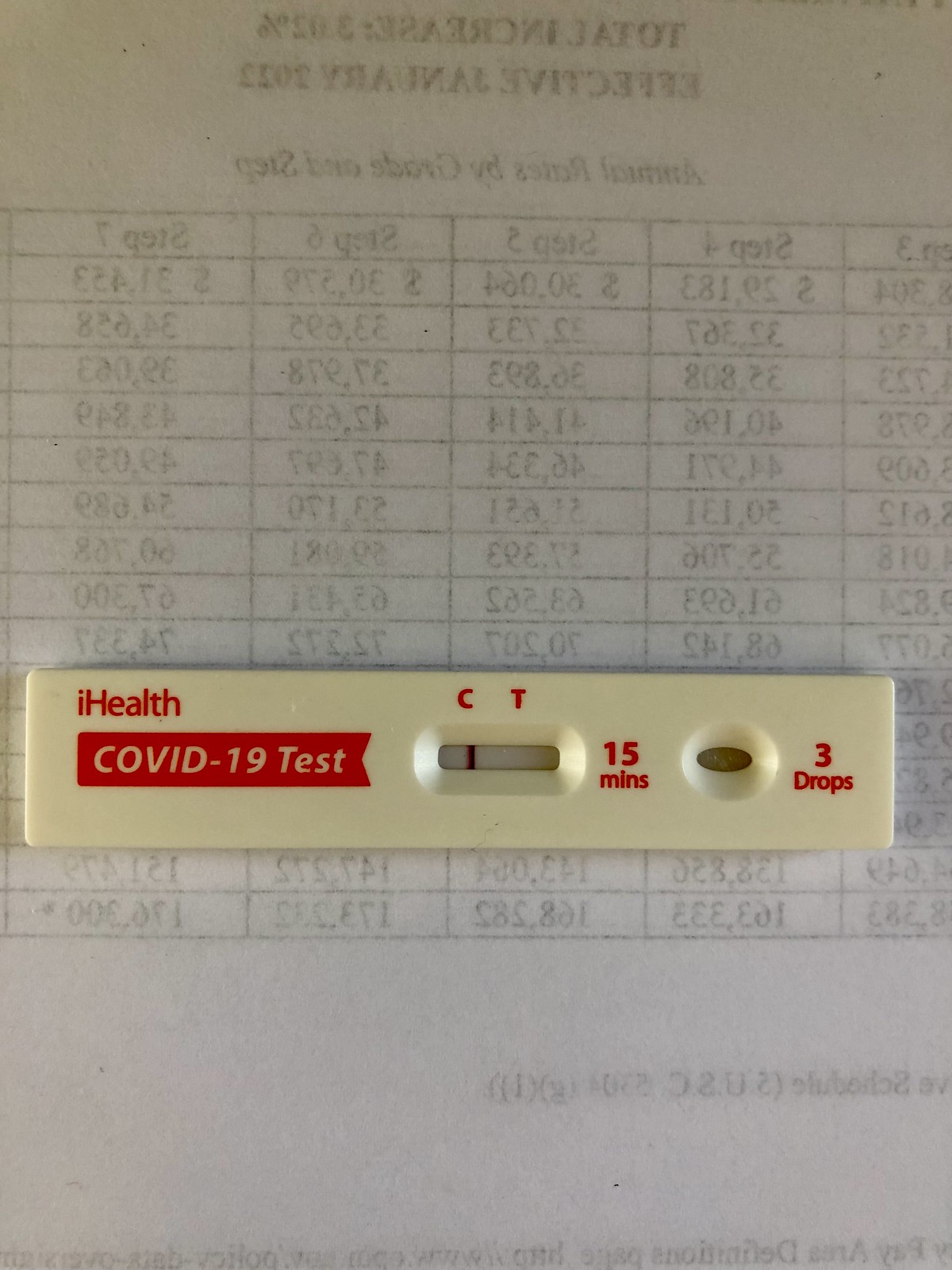A used COVID-19 rapid test sits atop a sheet of financial documents. The test has a single line in the control area, indicating a negative result. Three drops of the individual's nasal sample were placed into the designated sample well, as per the test instructions. The image captures the relief of a negative outcome amidst the backdrop of routine paperwork.